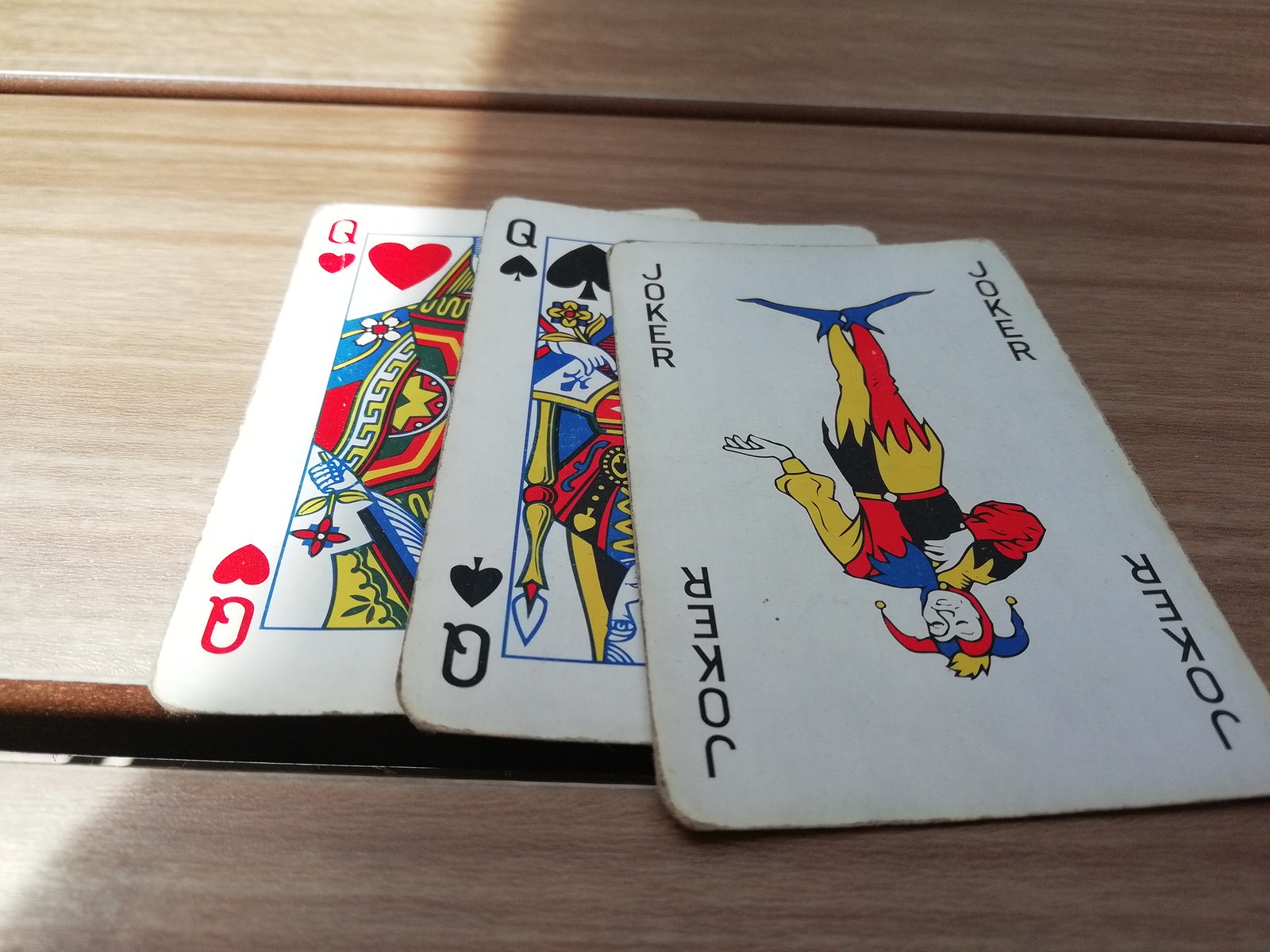A photograph captures a rustic wooden table with a light brown surface. Sunlight streams in from the left, creating a stark contrast with the shadows on the right side. The wood's surface features dark spots and small gaps between the planks, emphasizing its worn character. At the bottom of the image, there is a noticeable large dark gap where the table is slightly separated.

Placed prominently on the table are three playing cards: the Queen of Hearts, the Queen of Spades, and a Joker card. The Joker card is oriented upside down and features "JOKER" written in each corner. The Joker character depicted on the card wears a colorful outfit with red, yellow, and blue accents, blue pointy shoes, and a distinctive collar with blue and yellow trim. The figure's right arm is raised while the left arm extends sideways. The Joker's face is white with an exaggeratedly large nose, and they wear a whimsical hat adorned with blue, red, and yellow colors, accentuated with yellow tassels. The character is looking down, adding a playful, yet slightly mysterious, element to the scene.